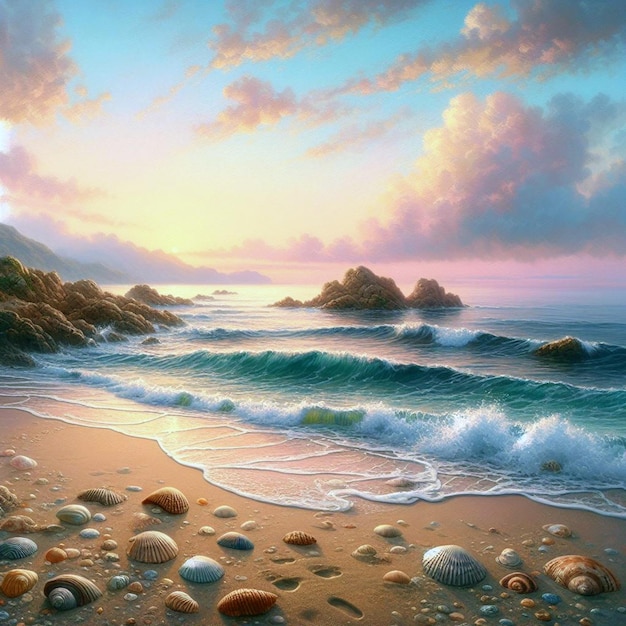The image is a square, AI-generated painting measuring approximately four by four inches, depicting a highly realistic beach scene rendered in an artistic drawing style. The foreground is dominated by brown sand studded with a variety of seashells, including clam, snail, and conch shells, as well as pebbles. Some faint footprints are visible among the shells. Three small, teal-green waves crowned with white foam crash gently into the shore. To the left and center of the painting, rocky boulders jut out into the water, adding texture to the seascape. The sky above is a mesmerizing display of a sunset, transitioning from pink and yellow near the horizon to purples and pinks among the clouds, eventually blending into a vivid blue at the very top. The overall effect is a stunningly lifelike yet clearly artistic representation of a tranquil, coastal twilight.